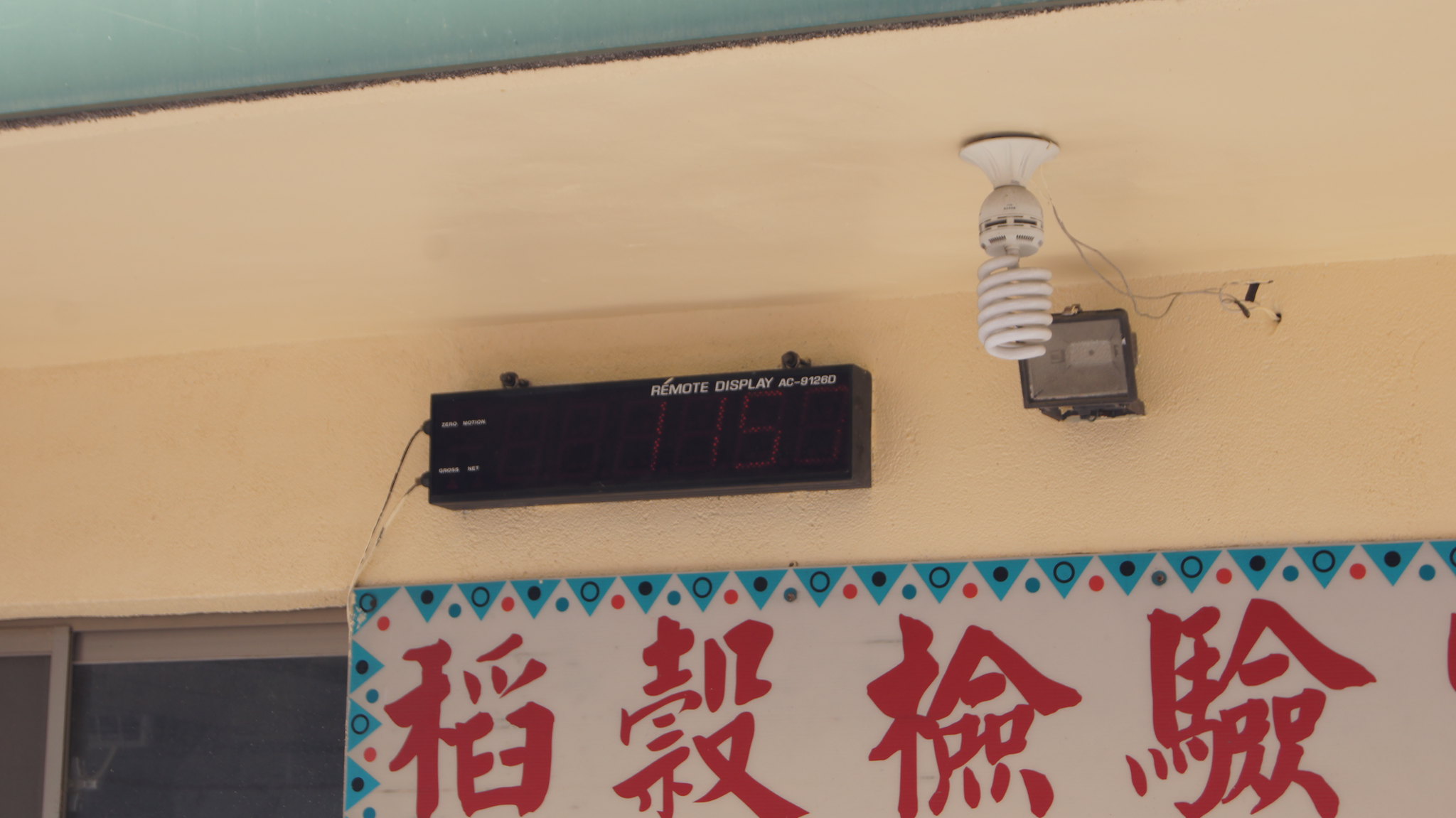The photograph captures a busy interior scene featuring a variety of elements. Central to the image is a black rectangular digital display mounted above a wall, labeled "remote display" with white font "AC-91280". The display is faintly showing the numbers "1150" or "115". The wall, painted in a warm off-white or light ivory color, hosts a white banner adorned with red Chinese characters and bordered with blue triangular patterns and alternating dots, both filled and outlined in black. Additionally, a bare coiled CFL bulb hangs to the right of the display, suspended from the ceiling by two cords. Adjacent to this light source, a square gray speaker is affixed to the wall. In the lower left corner, there's a glimpse of a possibly gray window or screen door. The uppermost part of the photograph reveals the ceiling in a light blue or teal color, creating a thin wedge shape above the wall.